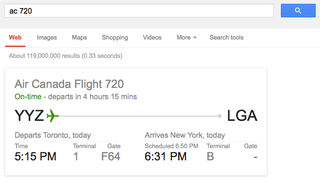The image is a screenshot of a web page displaying details about a flight within a web application. At the very top of the image is a long search bar containing the search phrase "AC 720." Directly below the search bar is a highlighted section with the word "Web" underlined in red. The main search results are displayed below this section, indicating approximately 118 million results. The top result features details about Air Canada flight 720, noting that the flight is on time and is scheduled to depart in 4 hours and 15 minutes. Below this, the airport code "YYZ" (Toronto Pearson International Airport) is displayed in black, accompanied by a green airplane icon. A horizontal gray line extends from this icon to the airport code "LGA" (LaGuardia Airport, New York) also written in black. Beneath "LGA," in gray text, it states, "departs Toronto today."